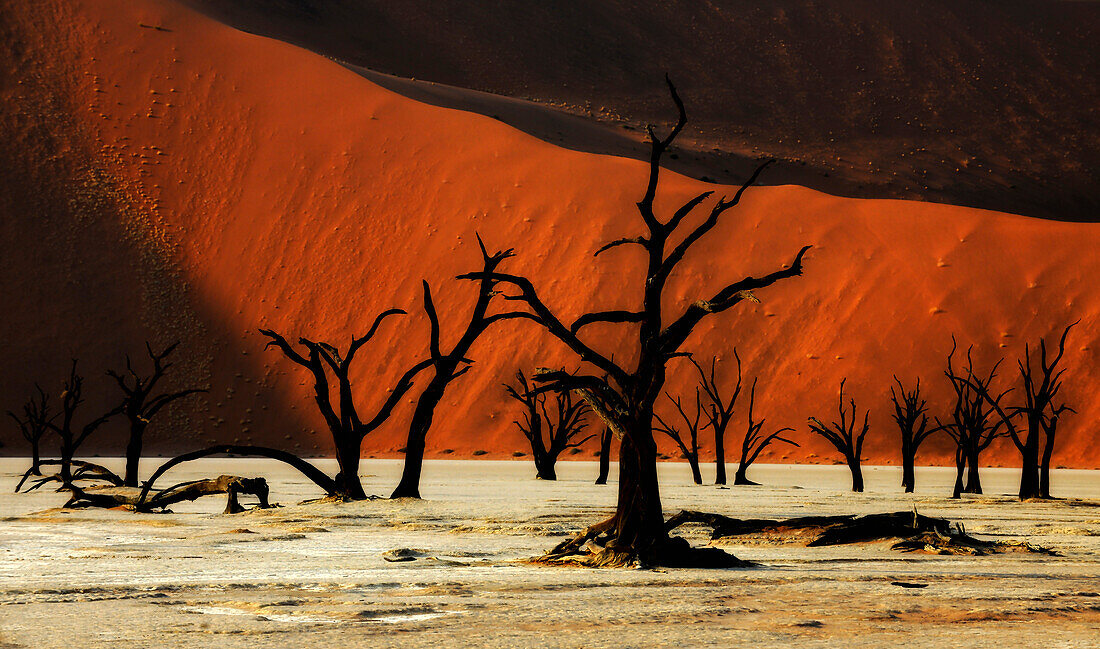This photograph captures a stark, desolate landscape, possibly a desert or a wasteland. The ground in the foreground is covered with light brown dirt and sand, devoid of vegetation. The main subjects are the barren, leafless trees, which appear scorched black as though by fire or extreme conditions, adding a sense of decay and abandonment. These trees show various stages of collapse, with some reduced to roots and others falling over, their spikes accentuating their lifeless state.

The midground features a massive, vividly bright reddish-orange sand dune, its surface marked by diagonal lines possibly caused by wind erosion. Sprinkled across the dune are small white specks, potentially rocks or other debris, and a larger cluster of these specks on the left side suggests a rock slide or exposed minerals.

In the background, the landscape transitions to a darker, almost ominous dark brown area, which might be additional mountain ranges or more sand dunes under a shadowy light, adding a dramatic contrast to the scene. The overall effect is a hauntingly beautiful, yet eerie image, capturing the raw and harsh beauty of what appears to be a lifeless, arid terrain.